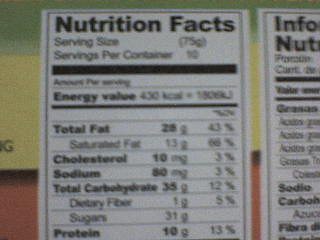A close-up image captures the nutrition facts table on a food container. The container features a vibrant design with horizontal stripes: green at the top, yellow in the middle, and red at the bottom. The nutrition label reveals that a serving size is 75 grams, with the container holding approximately 10 servings. Each serving contains 430 calories, 28 grams of total fat, 13 grams of saturated fat, 10 milligrams of cholesterol, and 80 milligrams of sodium. Additionally, there are 35 grams of total carbohydrates, which include 1 gram of dietary fiber and 31 grams of sugar. The protein content per serving is 10 grams. The compactness of the image makes the detailed nutritional information easily accessible and legible.